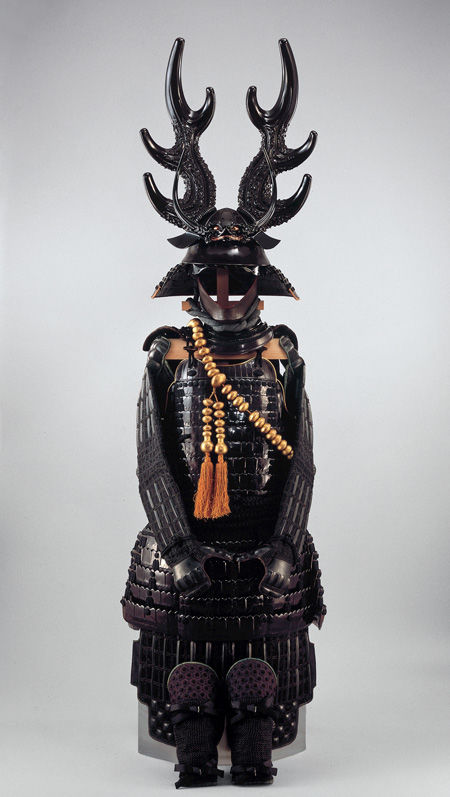The image showcases a hauntingly detailed statue, seemingly crafted from either dark-colored metal, hard wax or wood, representing an ancient warrior or a supernatural figure. The head features a prominent, mask-like visage devoid of facial features, crowned with an elaborate headpiece. This headpiece combines small, straight horns at the front and large, antler-like horns extending from the sides, echoing the majestic antlers of an elk. Draped across its shoulders is a distinctive gold braid adorned with red or orange tassels. The figure is clad in a highly stylized, predominantly black uniform with scattered brown tones, evoking the appearance of ancient armor with intricate scaling and shielding. The statue's overall attire includes a jacket with long, thin sleeves that hang empty, and large, armored boots that anchor the statue firmly. The central positioning and meticulous craftsmanship of this statue contribute to its eerie, yet captivating presence.